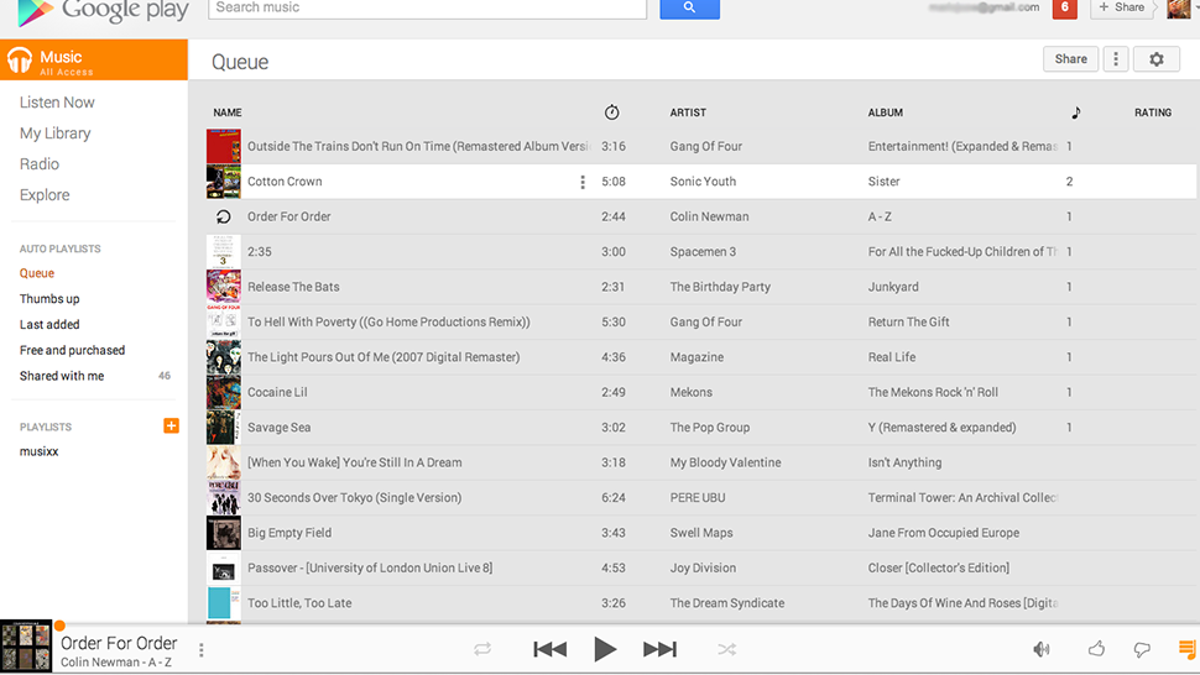This screenshot captures the Google Play interface featuring a light grey header. In the upper left corner, there is a triangular icon representing Google Play. Beside the icon, "Google Play" is prominently displayed in large grey text. Adjacent to this, a white search box displays the prompt "search music," accompanied by a blue magnifying glass icon. Moving to the far upper right, there's a red square with the number six in white, indicating notifications, and a barely visible user profile image.

To the left side, an orange banner with white headphones displays the word "Music." Below this banner, a vertical menu lists various options: "Listen Now," "My Library," "Radio," "Explore," and "Auto Playlists." It also includes several specific playlists and categories in orange text: "Queue," "Thumbs Up," "Last Added," "Free and Purchased," and "Shared with Me." The "Queue" item is highlighted on a white banner, and to its right are two icons in dark grey—a share button and a settings button.